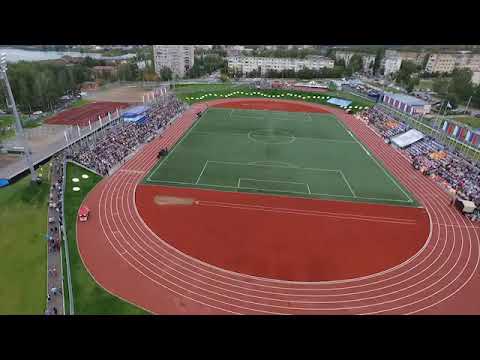The photograph presents an overhead view of a vibrant sports complex, with a green football field at its heart, encircled by a striking red running track. The image is captured from a high vantage point, offering a comprehensive view of the facility. Spectators fill the stands on both the left and right sides of the track, attentively observing the scene below. Despite the slight blur and distortion in the picture, the daytime setting is clear, as natural light illuminates the entire area. In the distance, beyond the stadium, buildings and trees form a scenic backdrop. Additionally, in the top left corner of the image, a glimmering water body can be spotted. Notably, two horizontal black strips frame the top and bottom of the photograph.